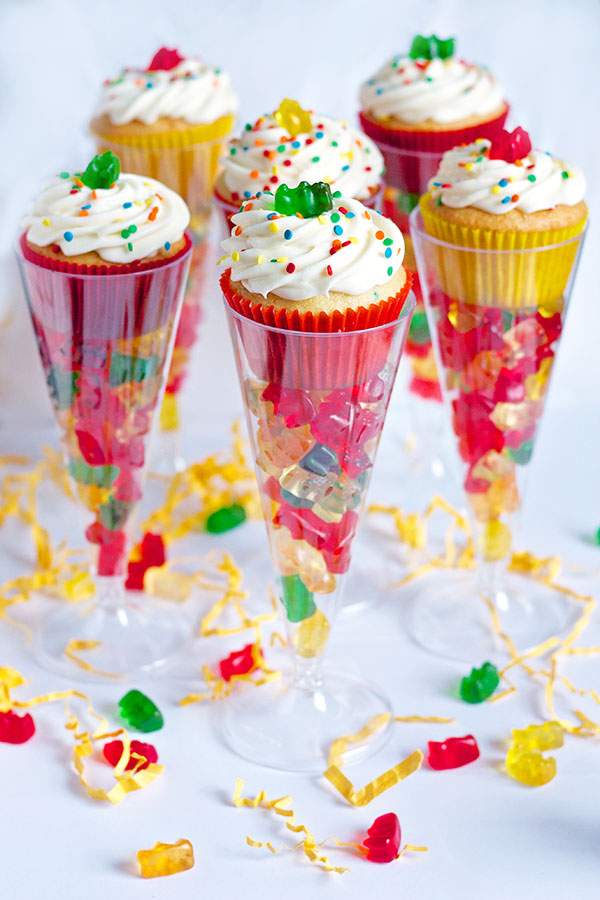This image showcases six vanilla cupcakes displayed in clear, cone-shaped champagne glasses. The glasses are arranged in a circular formation with five surrounding one in the center. Each glass contains a cupcake nestled atop colorful gummy bears, which match the scattered jelly beans around the setup. The cupcakes have white frosting sprinkled with tiny colored speckles, and each is adorned with a single jelly bean on top. The cupcake wrappers are in vibrant shades of red and yellow, and more gummy bears are visible beneath them inside the glasses. The composition is set against a pristine white background, accented with thin strands of yellow confetti scattered lightly. The vibrant gummy bears—red, green, yellow, and even some clear—add an extra festive touch, making the entire scene look like a delightful party favor or an inviting after-dinner dessert.